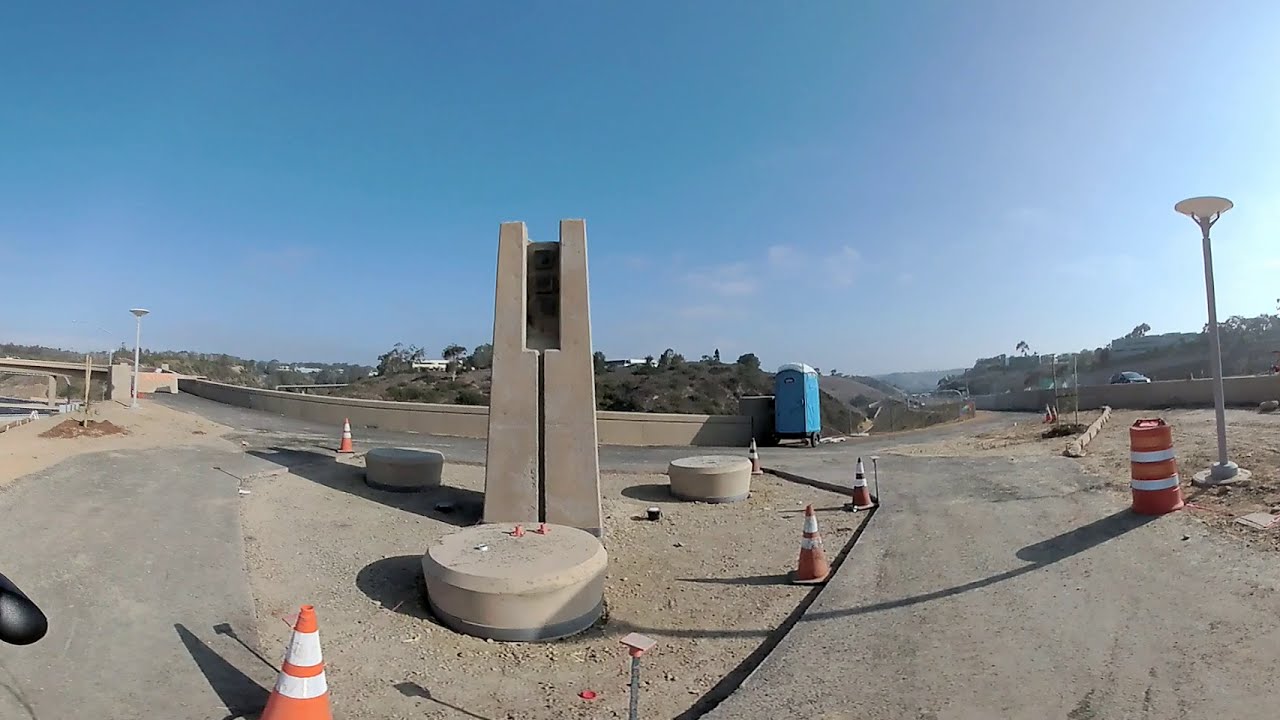This detailed image captures midday road construction of a new off-ramp by a freeway, featuring a newly paved asphalt road lined with several orange traffic cones with white tape near their tops. Central to the scene is a prominent stone structure resembling a monument or pillar, surrounded by three stone circles. On the right side of the image, a blue portable toilet on wheels is situated at the construction site’s corner. Cars are visible on the roadway, primarily to the right, indicating active traffic. To the left, beyond the freeway, a hillside is visible, and further back, a patch of land dotted with trees stretches across the background. The sky above is clear and light blue with only a few clouds, and the overall setting appears sunlit, suggesting a bright, sunny day that gives the landscape a somewhat desert-like ambiance, typical of a Californian environment. No text is present in the image.